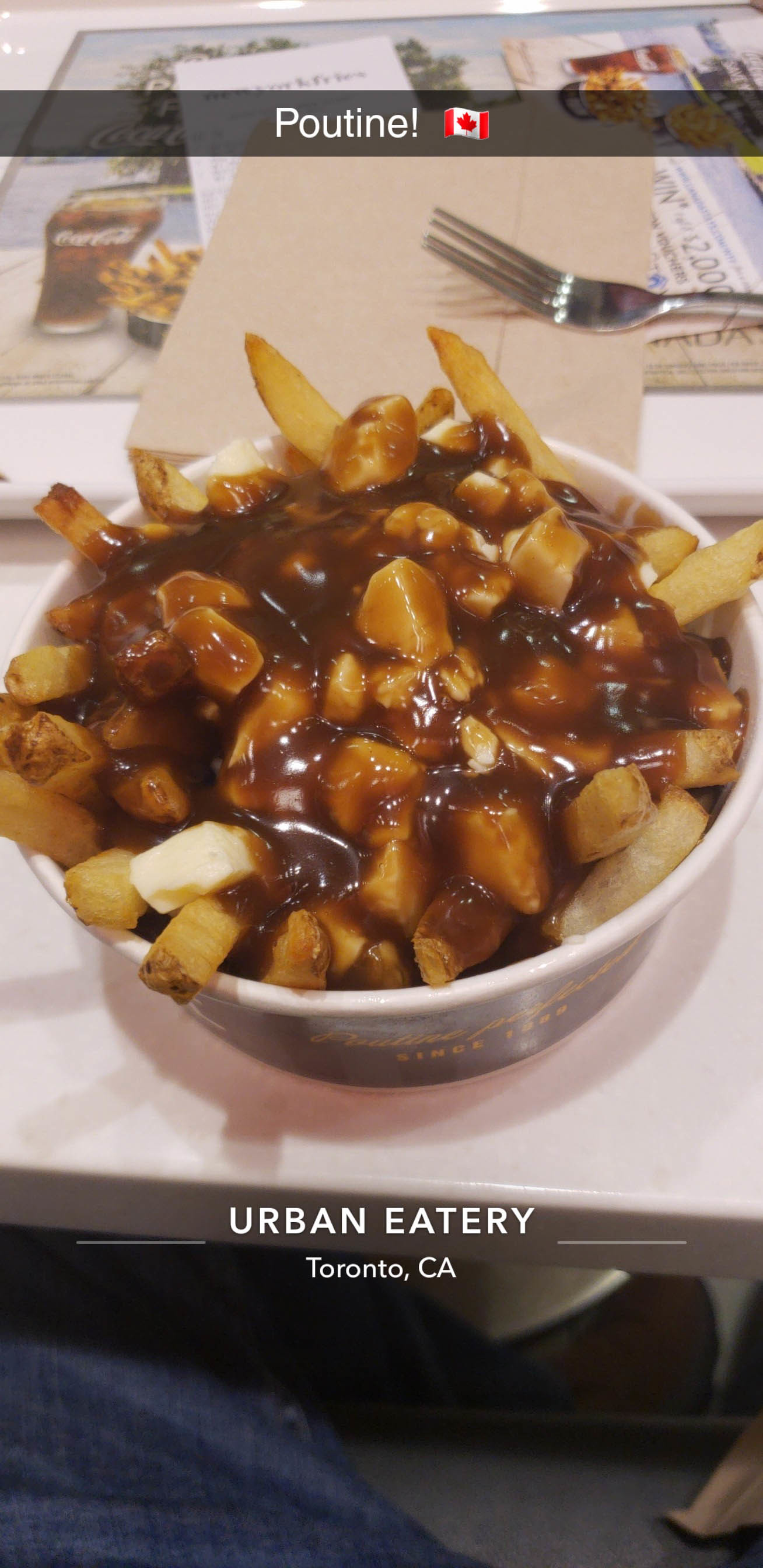This detailed indoor photograph showcases a meal setup at Urban Eatery in Toronto, Canada. Central to the image is a thick, round disposable bowl brimming with poutine, consisting of crispy french fries, white cheese curds, and glossy, dark brown gravy. A silver fork rests on a stack of brown napkins nearby. Above the bowl, a caption reads "poutine" accompanied by a Canadian flag, emphasizing the Canadian delicacy. At the bottom of the image, a caption indicates the location, Urban Eatery in Toronto, Canada. Scattered around the bowl are a receipt for the meal and an advertisement displaying various menu items including poutine and a cup of Coca-Cola. Part of a person's leg extends from beneath the table, adding a candid human element to the composition.